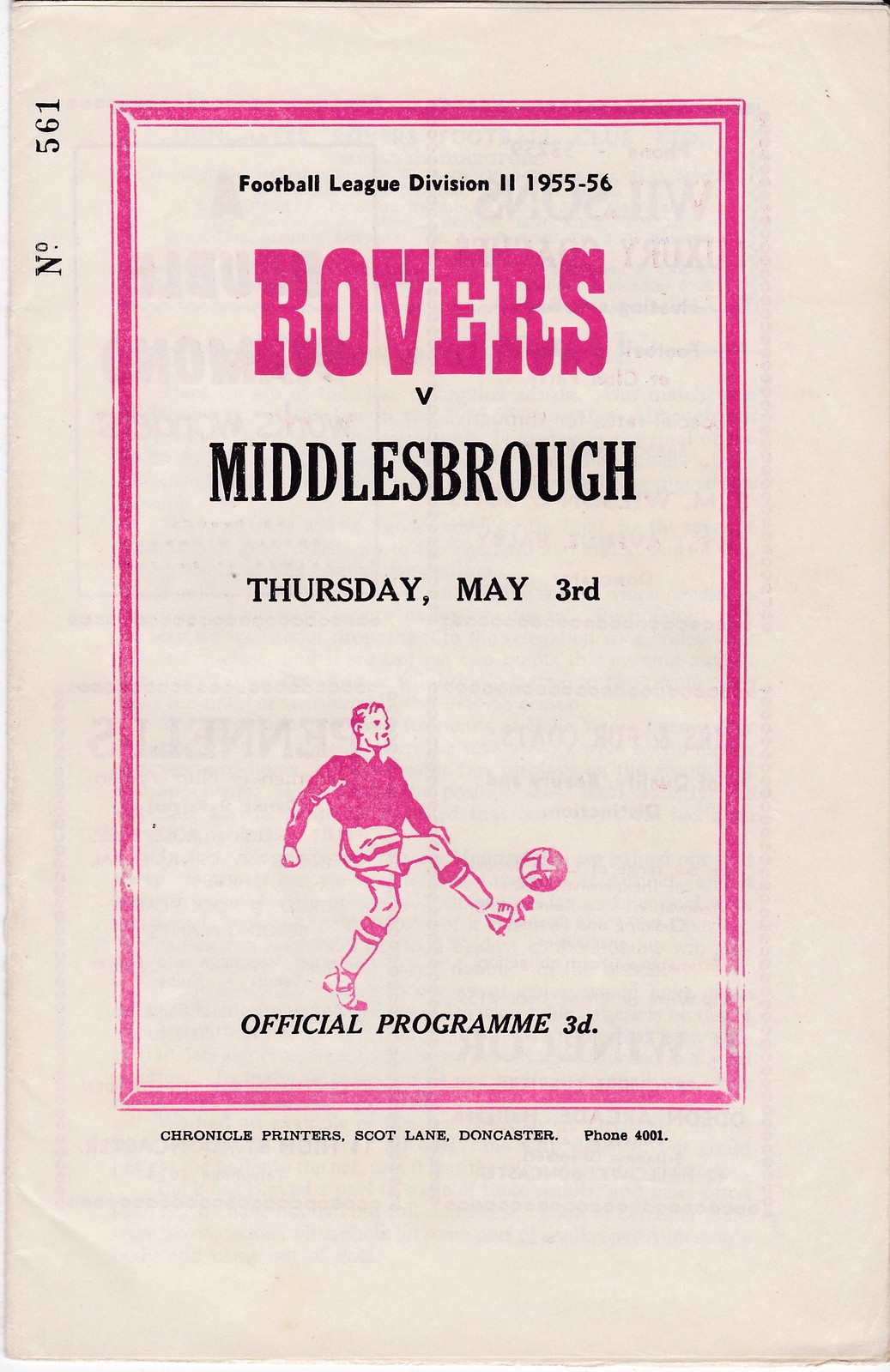This image is a rectangular cover of an old magazine or program, vertically oriented. The background resembles aged newspaper, off-white with subtle bleed-through from underlying pages. In the upper left corner, the number 561 is stamped vertically in black ink. Dominating the center is a faded pink rectangular border, enclosing text on a white backdrop. The black text within the pink border reads "Football League Division 2, 1955-56," and below that in bold pink letters, "Rovers versus Middlesbrough, Thursday, May 3rd." Further down, a pink illustration depicts a man kicking a soccer ball, with the caption "Official Program 3D" in black beneath it. At the very bottom, outside the pink border, small black text reads, "Chronicle Printers, Scott Lane, Doncaster, phone 4001." The cover shows signs of wear, with minor creases, adding to its vintage appeal.